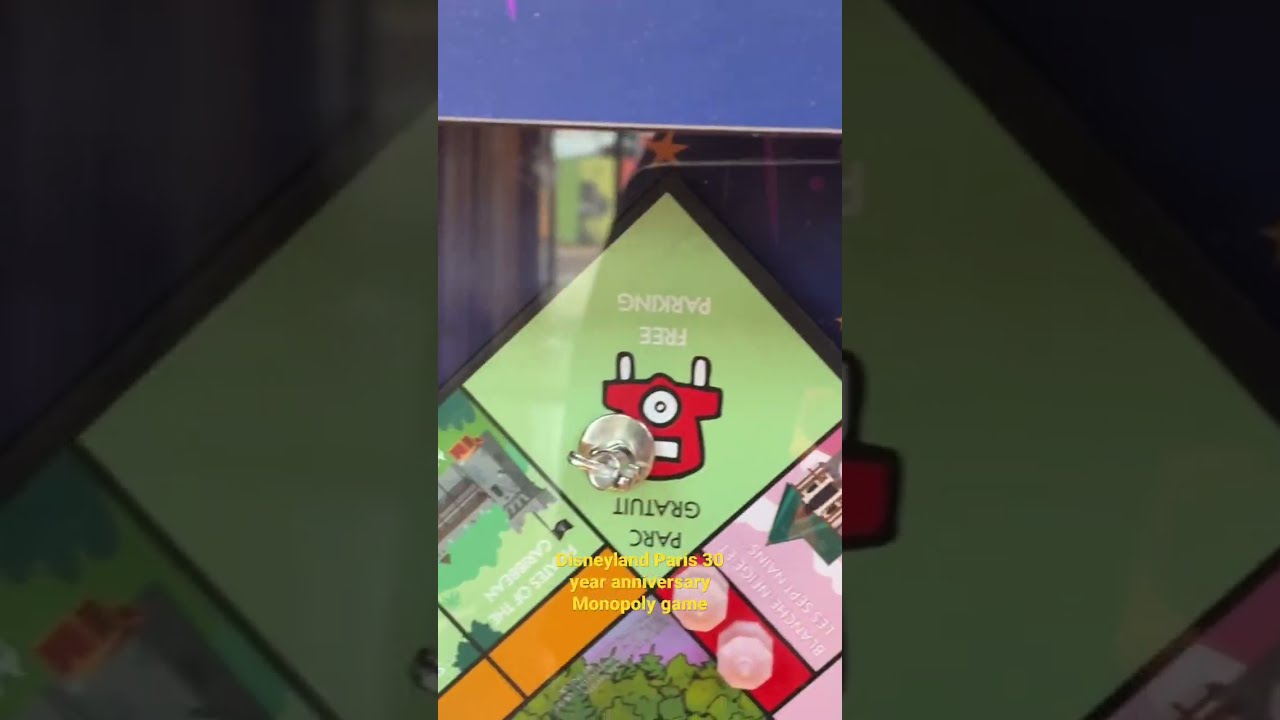This image features an open Monopoly game board designed for the Disneyland Paris 30-year anniversary edition. The board is positioned upside down on a glass table, with vivid blue, green, red, pink, orange, gray, and brown tiles. Central in the image is the Free Parking space, flanked by purchasable properties, including a castle and a Victorian-style house, indicating its thematic design. A game piece resembling a football helmet occupies the Free Parking space. Above the board, a darker blue border frames part of the image. Text stating "Disneyland Paris 30-year anniversary Monopoly game" is visible, highlighting its special edition theme. The background subtly reveals part of a room with an open window.